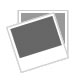This photograph captures an old comic book page resting on a concrete surface, with the edges of the surface visible. The comic book, printed on yellowed, white paper, looks very aged. It appears to be part of a stack of similar comic books. The primary image occupies the top of the page, with three smaller images side by side beneath it, depicting a warfare scenario. The scene shows soldiers in military uniforms and hard helmets, engaging in combat with guns equipped with bayonets amidst explosions. The large title text at the top reads "VICTOR," styled with red lettering outlined in white. A yellow horizontal bar at the top right corner states "Laughs Galore Inside with the Hammer Man," while a black circle nearby indicates the price as 9p. Below this, a yellow grenade icon marks the start of the comic strip, which is described as "a true story of men at war" by displaying intense battle scenes with soldiers moving forward amidst the chaos.